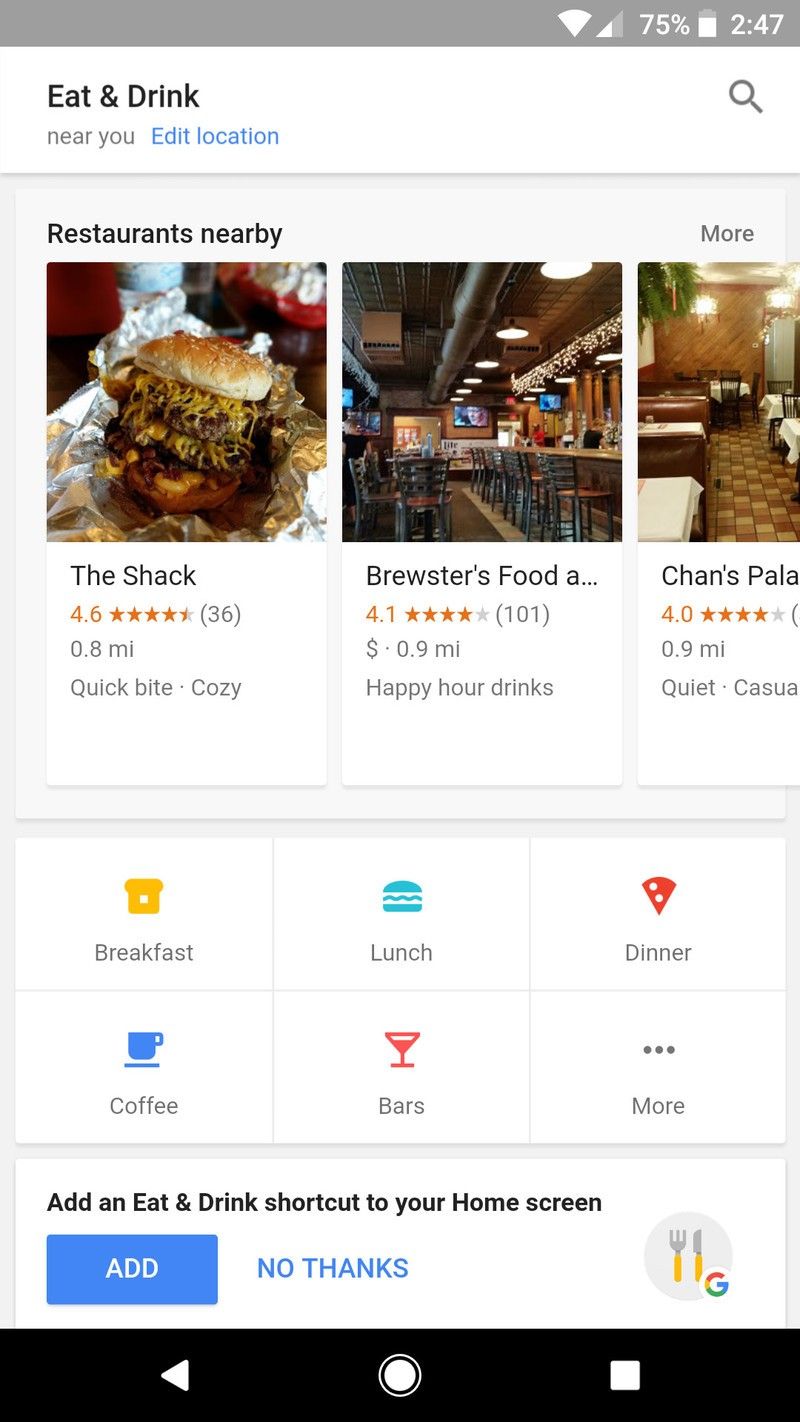This image displays a detailed view of a cell phone screen showcasing a list of nearby dining options. In the upper right corner, icons for wireless signal, cellular connection, and a mostly full battery indicate connectivity status, with the battery at 75%.

At the top of the screen, a title reads "Eat and Drink Near You" with an option to edit the location. Under this heading, there are three photos representing nearby restaurants:

1. **The Shack**: The top left photo is a close-up of a hamburger, likely triple-patty, stacked high with onions and what appears to be mustard spilling out. It is partially wrapped in tinfoil. Below the image, details read: "The Shack, 4.6 stars, 0.8 miles, quick, bite, cozy."

2. **Brewster's Food**: The middle photo depicts the interior of a bar. On the right side, a bar counter with chairs and a turned-on TV set in the background can be seen, while tables with chairs are situated on the left. The text beneath reads: "Brewster's Food, 4.1 stars, 0.9 miles, happy hour drinks."

3. **Chan's Pala**: The right photo shows the inside of a restaurant with a tile floor, featuring booths in the foreground and a table with chairs in the background. The partial text below it reads: "Chan's Pala..., 4.0 stars, 0.9 miles, quiet, casual."

Under these images are icons representing meal categories and beverages:

- A piece of toast icon labeled "Breakfast"
- A hamburger icon labeled "Lunch"
- A pizza icon labeled "Dinner"
- A coffee cup icon labeled "Coffee"
- A wine glass icon labeled "Bars"
- An icon with three dots labeled "More" 

This screen effectively provides a quick, comprehensive overview of dining options with corresponding visual aids and essential details.